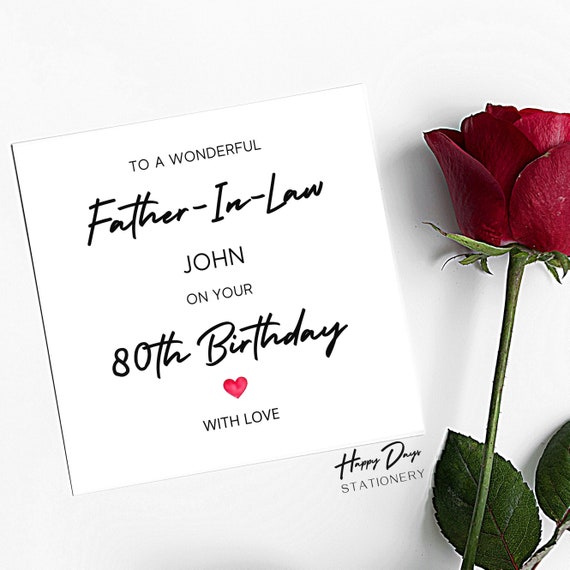This image depicts a birthday card for someone’s father-in-law named John on the occasion of his 80th birthday. The card itself is square and positioned slightly crooked to the left. It is set on a white surface, against a pure white background. The text on the white card is primarily black, with "father-in-law" and "John" written in a fancy font. The message reads: "To a wonderful father-in-law, John, on your 80th birthday," followed by a small red heart and the words "with love." At the bottom right corner, the card is branded with the text "happy days stationery". To the right of the card lies a long-stemmed red rose with a deep cherry red color. The rose is beginning to open and has small leaves underneath the partially visible blossom, with a slight imperfection on one of the petals.